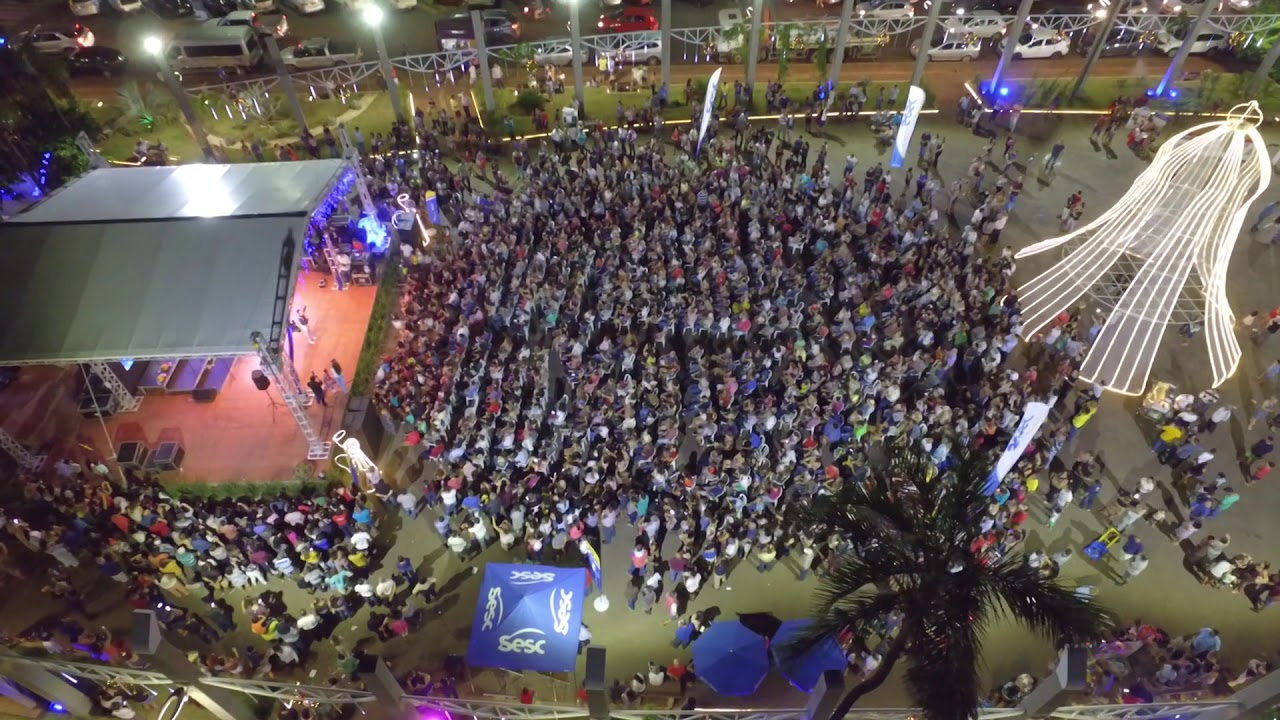The aerial photograph captures a lively nighttime concert scene with a large, enthusiastic crowd. Dominating the left side is an open-air stage with a distinctive red floor and a silver metal roof, where performers can be seen under the bright, non-natural lights of spotlights. Surrounding the stage, both in front and to the sides, are numerous concertgoers tightly packed together, with additional clusters beneath several blue awnings providing cover. On the right side of the image stands an illuminated white structure resembling a bell, adding a decorative touch to the event. The area appears to be enclosed, with various canopies and vendor coverings scattered about, as well as palm trees overhead. In the background, beyond a boundary, a roadway is visible lined with parked vehicles, flanked by what looks like storefronts and a grassy area, creating a lively, festive atmosphere.